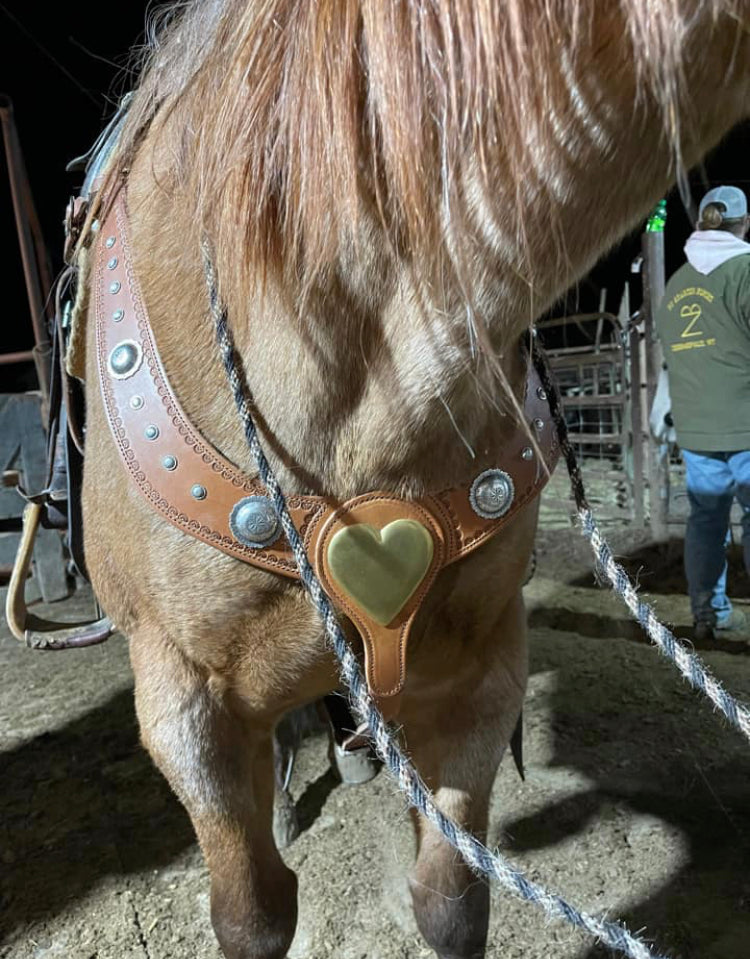The close-up image showcases a light brown horse, focusing on the intricately detailed mardingale that secures its saddle. This leather harness is adorned with numerous silver rivets, some of which feature intricate inlaid images. At the center of the horse’s chest, there is a distinctive gold-colored heart-shaped ornament. The harness also boasts decorative stitching. The horse's neck is draped with off-white and black striped ropes that hang down on either side. The stirrups, visible on the left, appear well-used but maintained. In the background to the right, there's a man wearing an olive-colored jacket with yellow writing and an emblem resembling a 'Z' with a 'B' on top, facing away from the camera. The horse’s lighter beige coat transitions to a more brownish hue towards its legs, and its long hair adds to its majestic appearance.